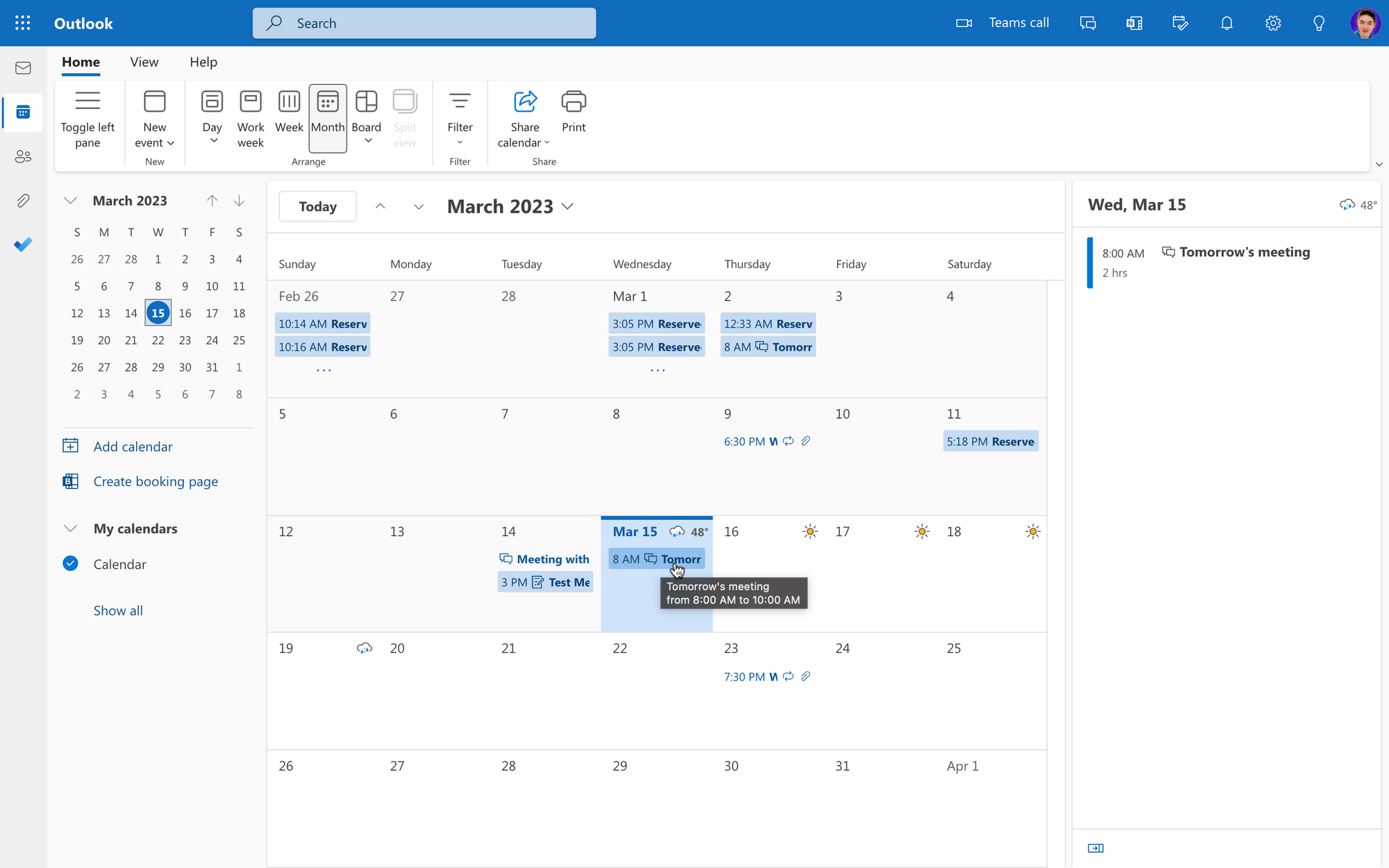The image is a horizontal screenshot likely taken from a computer or smart device, showcasing a digital calendar interface. The top of the screen features a long, attractive blue header bar. In the upper left corner, there's a grid icon next to the white text "Outlook." Adjacent to this, there is a light gray magnifying glass icon signifying a search bar. 

On the right side of the header, you'll find several functional icons: a Teams call icon, a bell icon, a settings icon, a light bulb icon, and a circular icon displaying a person's profile picture. The navigation menu along the top highlights "Home," which is bolded and underlined in blue. Other tabs include "View" and "Help."

Running vertically along the left side of the display are various icons representing different sections: email, calendar (this is highlighted), people, paperclip, and a blue checkmark. Below the "Home" tab, there are several options like "Toggle left pane," "New event," "Day," "Work week," "Week," "Month," "Board," "Filter," "Share calendar," and "Print."

The calendar view is set to March 2023, with a particular focus on March 15th, which is encircled and boxed for emphasis. The main portion of the image is taken up by the calendar itself, which is populated with various tasks and entries. To the right side of the calendar view, an event is detailed: "Wednesday, March 15th, 8 a.m., 2 hours, Tomorrow's meeting."